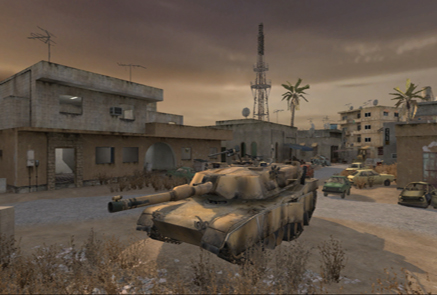This image is a computer-generated rendering, possibly from a video game, depicting a military scene. Dominating the center foreground is a tank with a tan and brown camouflage pattern. The turret, mounted on the rotating top part of the tank, faces towards the left. The tank is positioned diagonally, with its front facing left and the back facing the upper right. The vehicle's tracks are attached to the rusty-brown areas around the wheels, and it sits on lighter brown dirt, possibly part of a paved roadway.

Surrounding the tank are a mix of concrete buildings and low scrubby grass with tiny white specks, likely representing flowers. The buildings to the immediate left and behind the tank range from one to four stories tall, composed mostly of concrete with rectangular windows. A notable feature in the scene is a large metal tower and several TV antenna-like structures on top of the buildings. The tallest building in the center has arched top windows and a communication or radar dish on its roof. Additionally, there are a few old-looking cars parked around a four-story white residential complex on the right.

The background atmosphere is dark and stormy, with a very cloudy, gray sky and low cloud cover. Among the buildings, a large palm tree stands out next to the metal tower, adding to the war-torn and desolate ambiance of the scene.